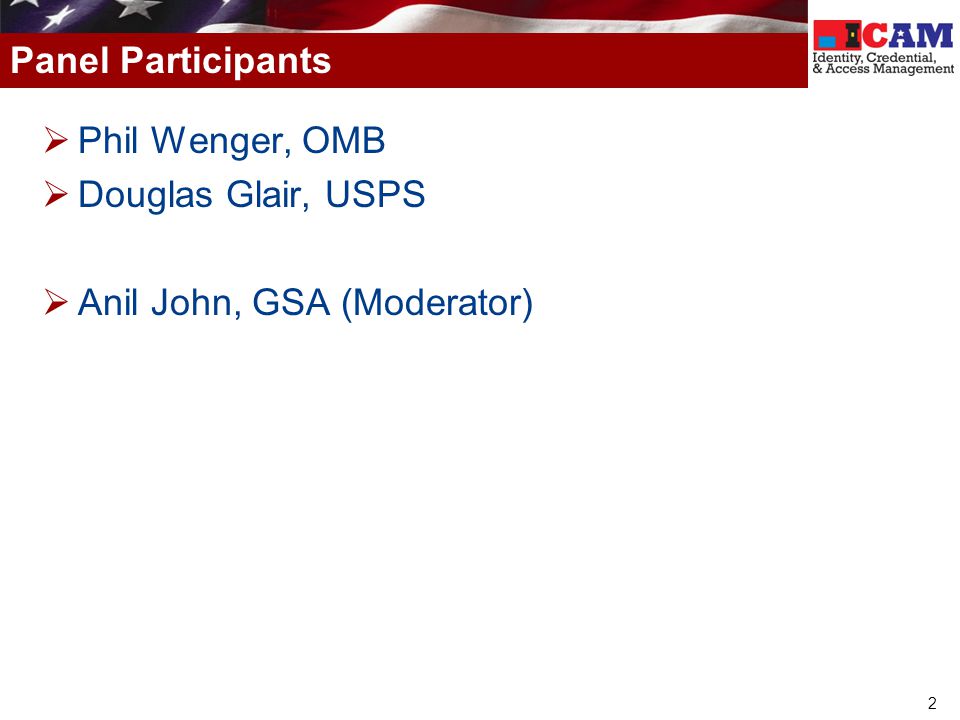The image is a horizontally rectangular graphic with no borders, featuring a prominent horizontal red stripe at the top that contains the text "Panel Participants" in white letters on the left. To the right of this text, there is a colorful logo with the letters 'ICAM' where the 'C' is red, and the 'A' and 'M' are black, accompanied by the smaller text "Identity Credential and Access Management" beneath it. Below this header, three bullet points are presented using arrow graphics that point to the names of the panel participants, all written in blue text on a white background. The first name listed is "Phil Wenger, OMB," followed by "Douglas Glare, USPS," and finally "Anil John, GSA (Moderator)." Additionally, a segment of the U.S. flag is displayed above the red stripe, adding to the patriotic theme of the conference layout.